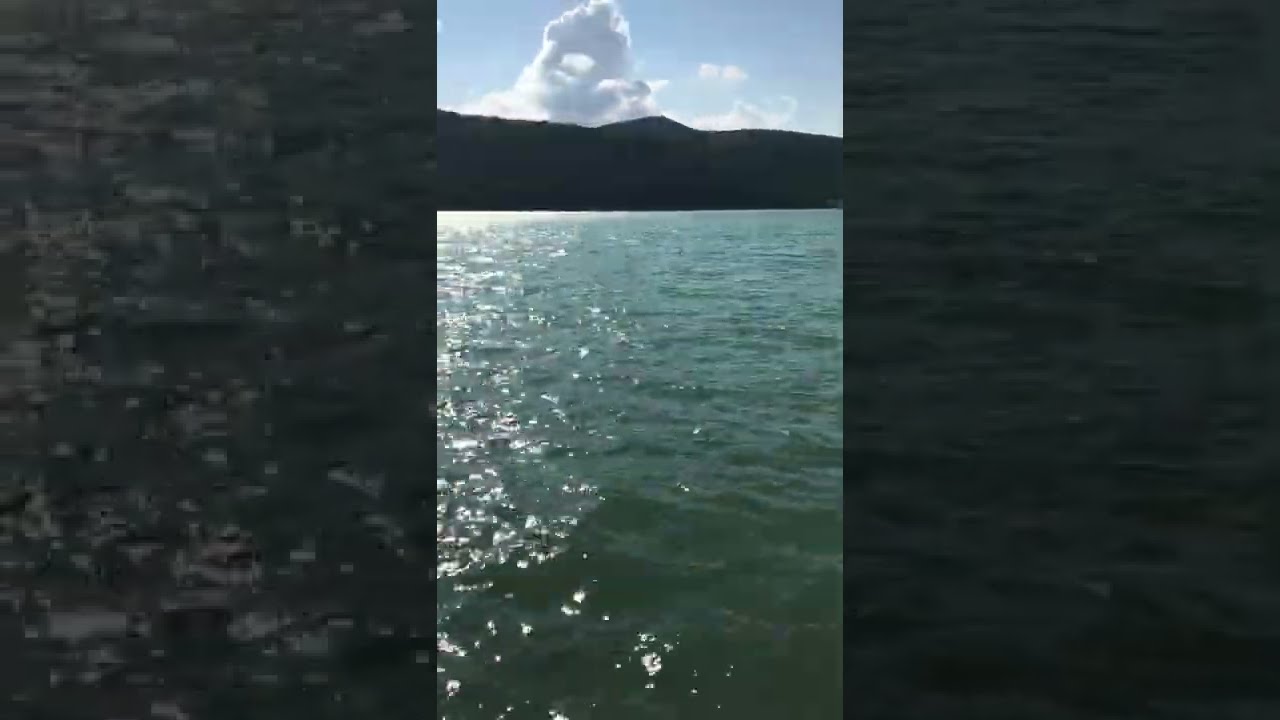This is a detailed photograph captured in vertical format, showing a serene and expansive body of water with a mesmerizing blend of teal blue and green hues. The water's surface shimmers, reflecting sunlight prominently on the left side, creating sparkling white glimmers, while the right side maintains a deeper, more subdued turquoise shade dotted with gentle ripples. In the distance, a vast mountain range rises, characterized by lush greenery and a mix of gentle slopes and a sharper peak in the middle. Above the mountains, the sky is a striking blue, punctuated by a scattering of fluffy clouds that transition from dark gray at the top to whiter shades at their bases. The daylight enhances the vibrant colors and tranquil atmosphere of the entire scene. There’s also a hint of a small, indistinct object in the far distance that might be a boat, adding a subtle point of interest to the expansive natural landscape.